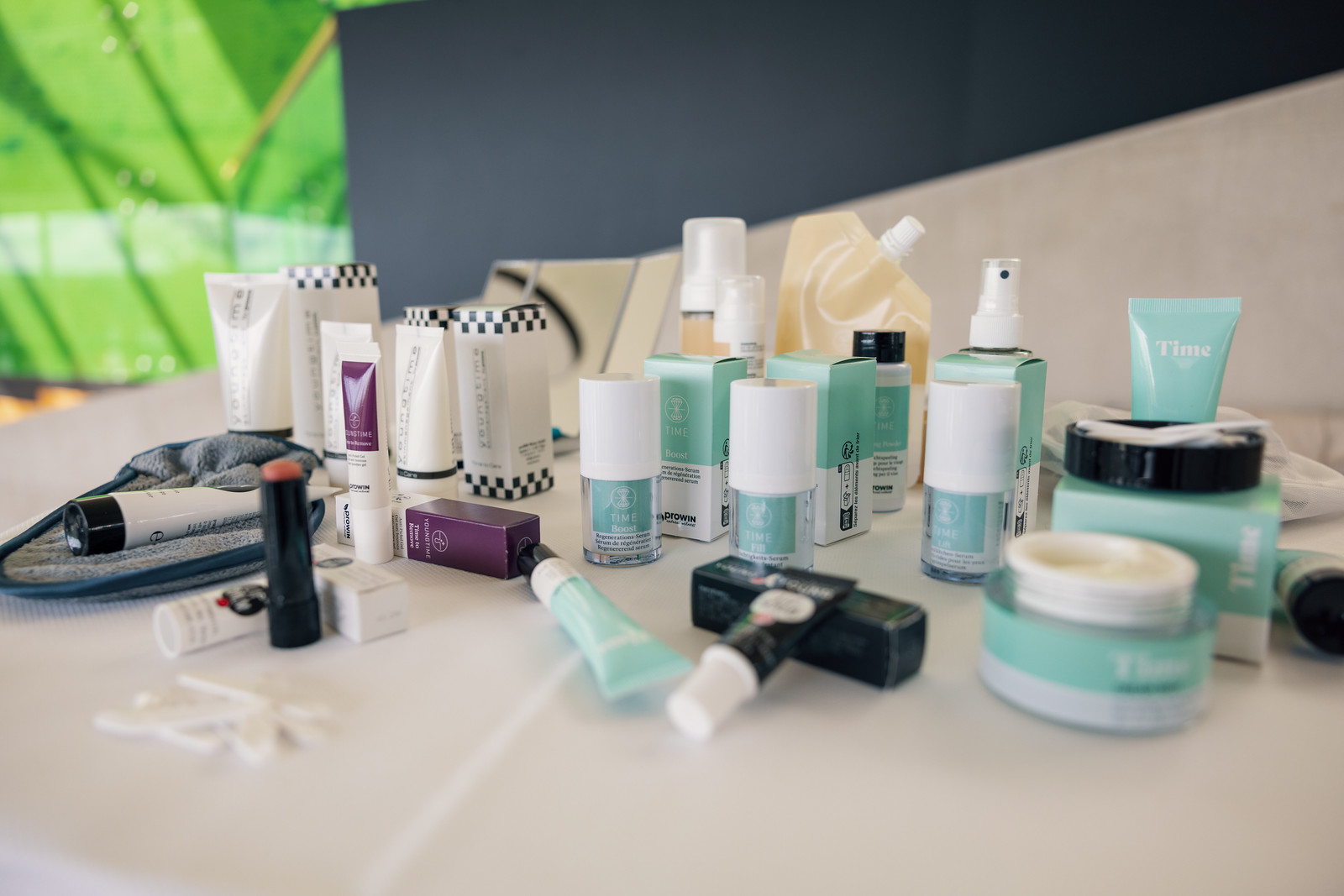This photograph captures the surface of a dressing table adorned with an array of makeup products, meticulously spread out for display. Predominantly, the items belong to the brand "Time," identifiable through visible logos and distinct packaging designs, although much of the fine text remains too small to be readable. The composition of the scene renders the farther objects slightly out of focus, enhancing depth perception.

In the foreground, we notice an unidentified tube of lipstick in shades of red and pink. A small gray sack occupies the left side of the image, potentially serving as either a storage bag or a sleep mask, with several makeup tubes resting atop it. The background reveals a dark gray wall on the right, juxtaposed with a vibrant green area to the left, enhancing the visual dynamics of the scene. An off-white wall harmoniously contrasts with the off-white tabletop, creating a muted yet elegant setting. The assortment features various makeup products, including sprays, tubes, lipsticks, and a jar with a screw-off lid, all arranged neatly on the off-white surface, showcasing the brand "Time."